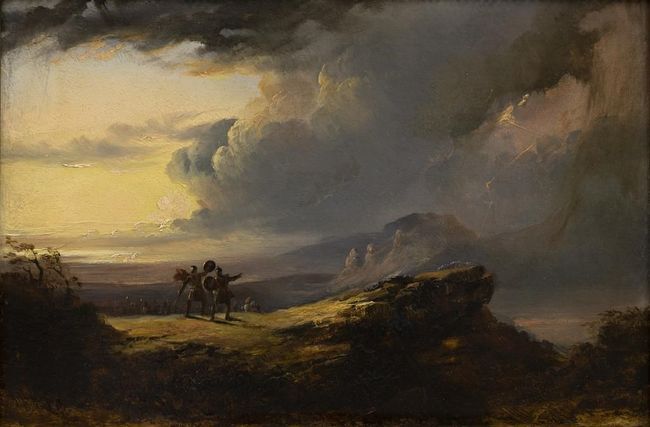This painting depicts a dramatic and somewhat ominous scene dominated by dark gray, rolling clouds that cover most of the sky. Towards the left, there is a break in the clouds, revealing some yellowish light, giving the impression of twilight or an approaching storm. The landscape features a rugged rock formation, primarily in shades of gray and brown, with a flat, golden-colored surface at the bottom of the painting. Two warriors, clad in tunics and holding shields, stand prominently on this rock, orienting towards the upper right, as if pointing at or anticipating something in the sky. Their presence suggests an air of readiness or foreboding, as they appear to be on the lookout. The background includes scraggly trees and additional dark rock formations, contributing to the overall moody and dark atmosphere of the scene. The painting effectively uses light and shadow to create a sense of depth and tension, aligning the brighter left side with a hint of hope or impending change against the darker, more oppressive right side.